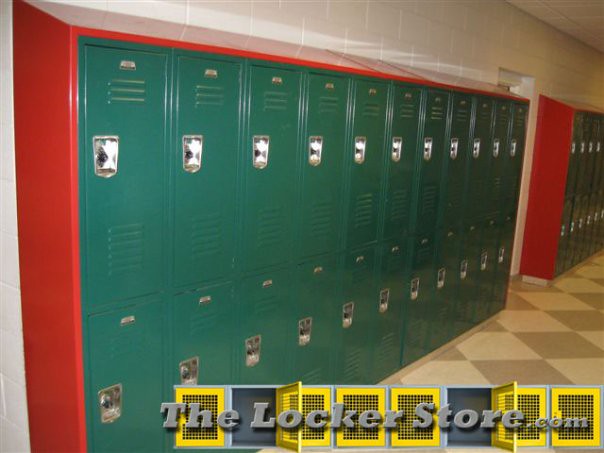In this image, we see a school-like setting with two large banks of green metal lockers, each outlined with a red trim and featuring silver handles. The lockers are arranged in two rows, creating a stacked effect. The photo is taken from a slight angle, causing the lockers to converge towards a vanishing point as they extend from left to right. The first bank of lockers visibly includes 22 lockers—11 above and 11 below—while the second bank partially visible due to the perspective, appears to have a similar arrangement. 

The lockers are set against a whitewashed brick wall, and the flooring below them is a checkered pattern of light beige and tan diamonds. At the bottom of the image, there is an advertisement for "thelockerstore.com" written in grey lettering. Behind this text, the logo features eight yellow locker doors with a mesh design within a blue frame, two of which are open (the second and the sixth lockers). This detailed composition suggests that the image is a promotional piece for a locker system by thelockerstore.com.